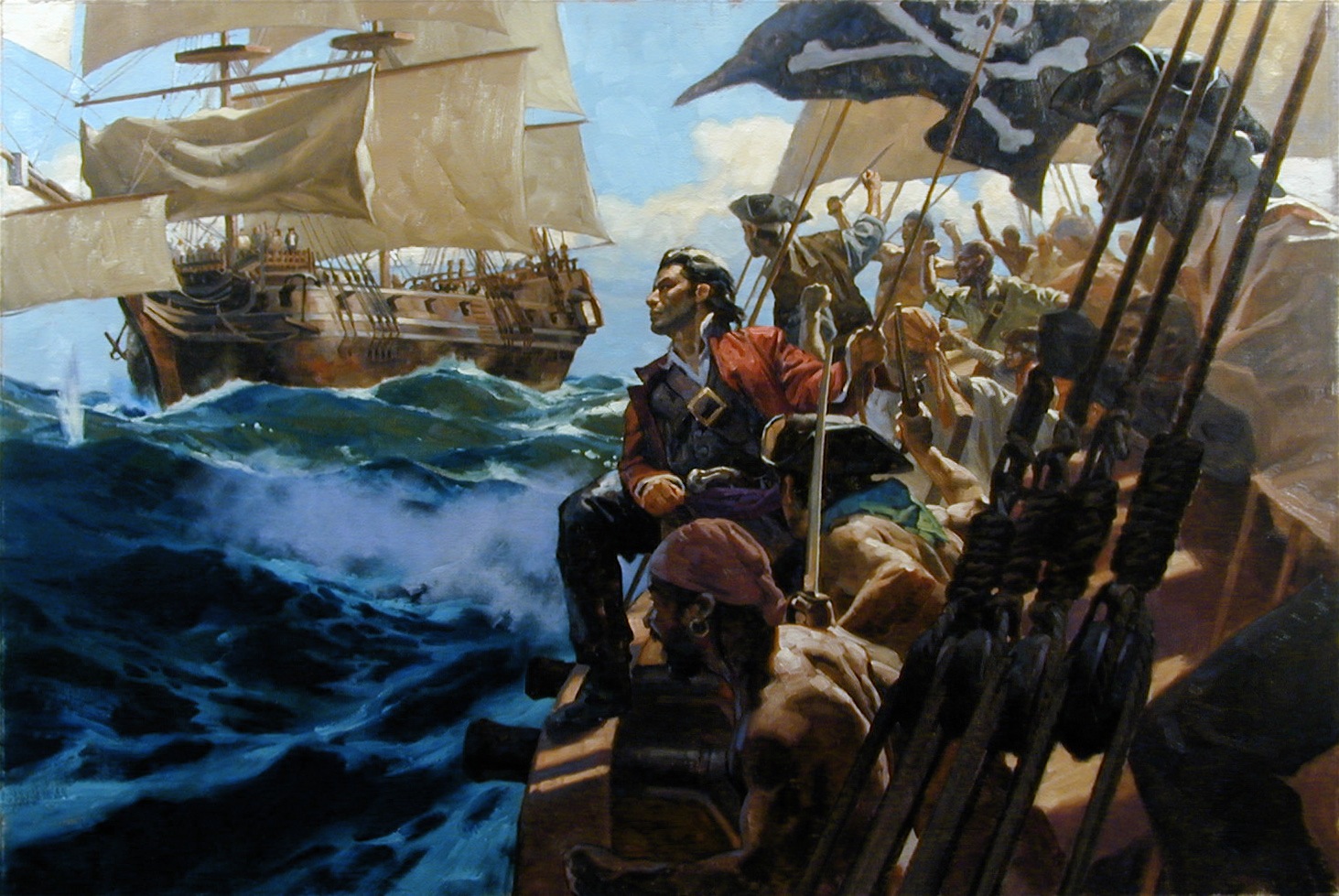This detailed painting, most likely an oil painting, depicts a daring scene of classic pirates preparing to intercept a large sailing ship on a turbulent ocean. The pirate ship occupies the foreground, its menacing presence amplified by the ominous Jolly Roger flag fluttering in the wind. The rigging is a labyrinth of ropes and pulleys, adding to the authenticity of the scene. A notable pirate, wearing a bandana and a gold earring, brandishes a sharp cutlass aloft, ready for combat. Another pirate, with a swashbuckling demeanor and a sash, joins the fray, also armed with a cutlass. The deck is teeming with activity as at least half a dozen more pirates, some wearing hats and others with bandanas, prepare for battle. Intriguingly, an African American pirate, distinguished by a black tricorn hat, is prominently featured in the right foreground, adding an uncommon historical element. The sea is depicted as rough, with large crashing waves enhancing the sense of imminent action. In the background, a three-masted schooner with full sails approaches, manned by sailors who are visible on both the foredeck and back deck. This ship, primarily wooden with a white flag, stands in stark contrast to the pirate ship. The stage is set for a dramatic confrontation as the pirates gear up to attack and board the approaching vessel, their readiness palpable.